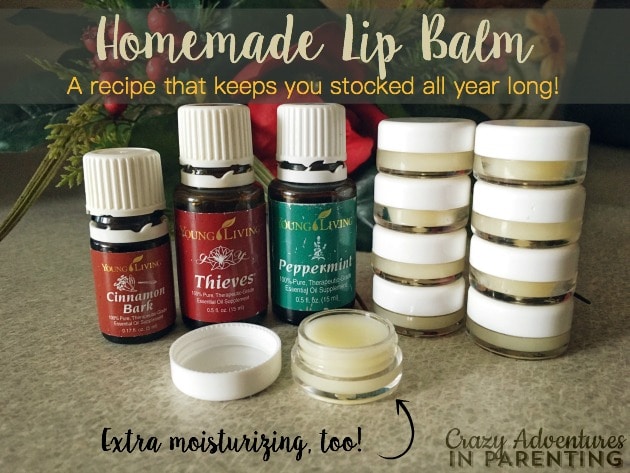This image is an advertisement for homemade lip balm that prominently features essential oils and is styled to resemble content from a parental blog. The advertisement is titled "Homemade Lip Balm: A Recipe That Keeps You Stocked All Year Long," and includes additional text such as "Extra Moisturizing Too" and "Crazy Adventures in Parenting."

The photo displays three bottles of essential oils—labeled Young Living Cinnamon Bark, Young Living Thieves, and Young Living Peppermint—each differing in size. To the right of these essential oil bottles are two stacks of four homemade lip balm containers, each with white caps.

At the center of the image is a single open lip balm with its cap placed to the left. The setting appears to be on a granite or table surface with colors prominently including red, green, white, orange, and black. The entire image is designed to imply the homemade lip balm is both practical for year-long use and particularly moisturizing, appealing to parents looking for natural, homemade skincare solutions.